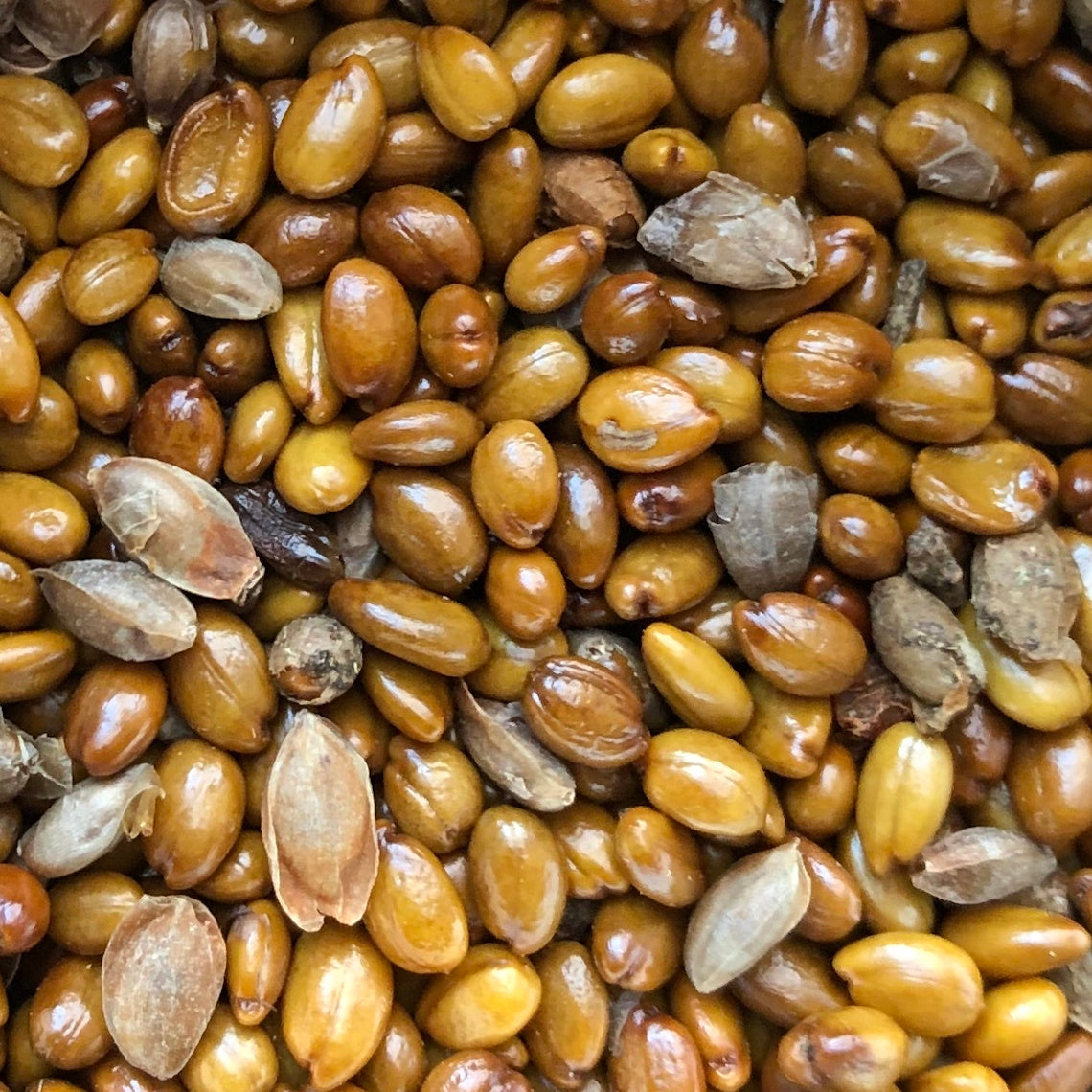The image depicts a close-up of a large, somewhat amorphous pile of cacao-like seeds or nuts, all varying in shades of brown from light golden to dark brown. The majority of these seeds have a shiny surface, reflecting light and giving them a polished appearance, while a few still retain their rough, dried husk. Flakes of these outer shells are visible, especially towards the top right of the image. The texture and colors range significantly among the pile, with some seeds appearing almost black and dried out. The focus is solely on the seeds, as there is no discernible background or foreground, adding to the depth and concentration of the pile. The bottom portion of the image is somewhat blurry, whereas the top is clearer, enhancing the details of the variety and condition of the seeds.